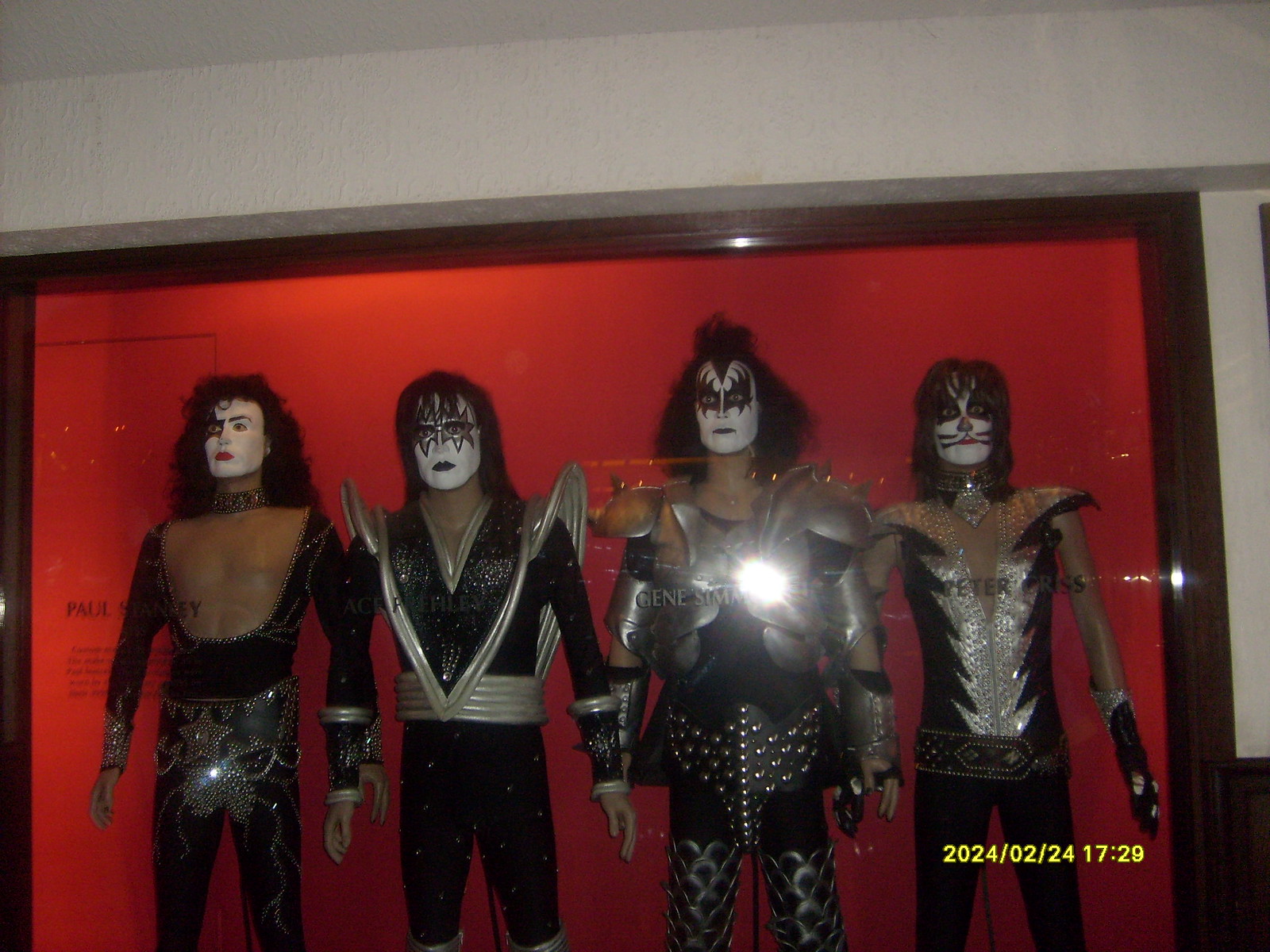This photograph, shot on February 24th, 2024, at 17:29, showcases a museum display featuring lifelike mannequin mock-ups of the iconic rock band KISS. Encased in a medium to dark brown wooden frame and backlit by a vivid red backdrop, the detailed mannequins stand inside an alcove covered by glass, reflecting light from the camera’s flash. Each figure dons the band's signature black and silver stage costumes that resemble armor or space-themed bodysuits, complete with sequined shoulder pads and elaborate belts. Their faces are painted in the distinctive white and black makeup styles that each KISS member is known for, some featuring bat-wing designs around the eyes, and varied designs such as a cat or a skeleton. With long, curly black hair styled to match their on-stage personas, these realistic replicas capture the essence and theatricality of the band's concert image.